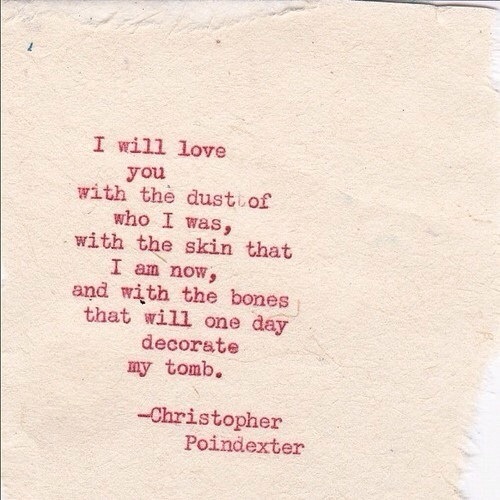This image features a short poem typed in red ink on light pink, handmade paper, characterized by a fibrous texture and jagged edges that lend it a vintage feel. The poem reads, "I will love you with the dust of who I was, with the skin that I am now, and with the bones that will one day decorate my tomb." It is authored by Christopher Poindexter, whose name appears neatly below the poem. The paper, seemingly delicate with visible threads along the sides, rests atop a piece of white paper, parts of which are visible especially towards the top and lower sides. The emotive poem speaks of a timeless and enduring love, encapsulating a sense of unfulfilled longing and devotion that extends beyond the poet's lifetime.